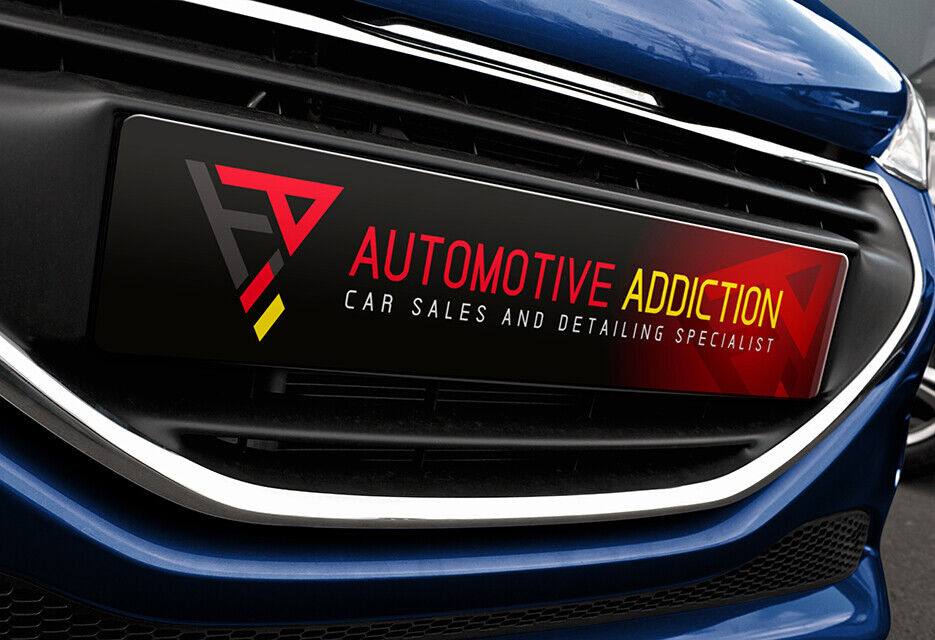This image is a close-up of the front of a blue car, capturing extreme detail and showcasing its glossy, shiny surface with reflections of clouds. In the center of the picture is a license plate area, but instead of a typical license plate, there's a sign with the text "Automotive Addiction" prominently displayed. "Automotive" is in bold red and "Addiction" is in bold yellow, both in all caps. Beneath this, in a smaller white font, are the words "Car Sales and Detailing Specialist." To the left of the text is a company logo, which consists of a red 'A' tilted at a 45-degree angle, a small yellow mark beside it, and some black line work underneath. The chrome grill and a headlight are visible on the right side of the image, against a backdrop showing gray concrete and possibly a wall. The setting appears bright, emphasizing the vehicle's gleaming exterior.